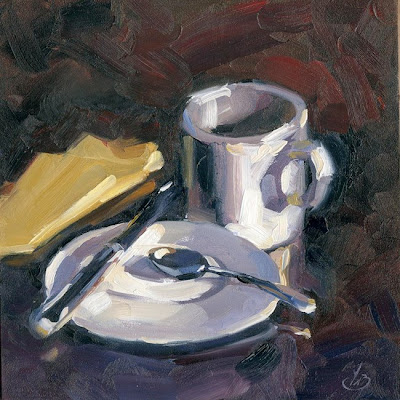This artist's painting vividly portrays a white plate with a silver spoon and a silver knife laid upon it, coupled with a white mug positioned up and to the right. The handle of the mug points in the same direction as the spoon's handle, and it boasts a wide brim with space enough for two fingers. To the left of the mug, there are two yellow objects, possibly napkins or slices of cheese, positioned in a stack. The background of the painting features a hodgepodge of colors—orange, red, yellow, green, white, purple, and pink—applied with distinct brush strokes, creating an abstract and distorted effect, almost like viewing through the bottom of a glass. This background, void of any people or text, contains the subtle initials of the artist, perhaps "T.A.," encircled in a semi-circle at the bottom right. The overall composition is somewhat indistinct and abstract, inviting interpretations through its play of color and form.